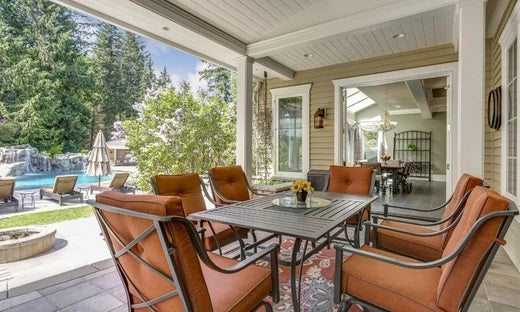This image depicts a covered patio area at the back of a residence, showcasing an outdoor dining setup and a scenic backyard. At the center of the patio is a large dining table constructed of pewter-colored metal with slotted design, accompanied by six matching captain-style chairs. The chairs feature upholstered orange seats and orange pillow backs, adding a pop of color to the setting. On the table, there is a small vase containing yellow sunflowers, adding a touch of natural beauty. 

The patio is characterized by white columns and a white ceiling overhead, giving it a spacious and airy feel. Underneath the table, there is an oriental rug in shades of orange and gray, placed atop tan pavers that cover the patio floor. To the left side of the image, we can see a swimming pool surrounded by lounging chairs and a pool umbrella. Between the patio and the pool lies a fire pit constructed from tan stones. The background is framed with tall trees, enriching the overall serene ambiance. Beyond the open patio door, the interior of the house is partially visible, displaying another dining area complete with a chandelier.